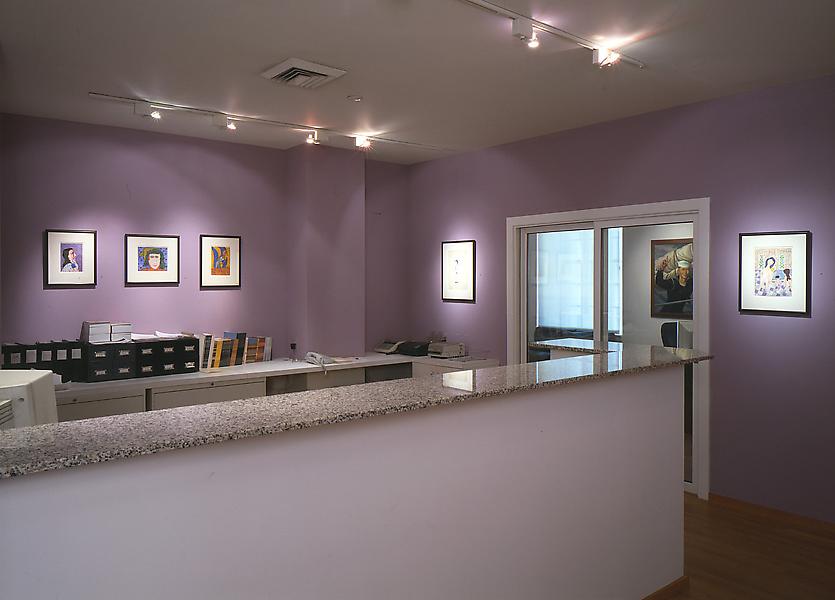This image depicts a professional office setting, potentially a dentist’s office, characterized by its light purple walls and wooden flooring. A prominent white counter with a granite, or marble-like, black and white top dominates the foreground. Behind this counter sits a computer monitor, noticeable for its bulky, possibly 90s-era design, alongside a telephone to the right. The back of the office features an organized filing system with black binders and an open-shelf cabinet. A row of books and what appears to be a note card system, reminiscent of old library catalogs, is visible as well. In the corner, an unidentified electronic device, potentially a fax machine, stands out. Above, the ceiling hosts several rows of lights, a vent, and two sliding glass doors that likely lead to another room, quite possibly a conference room. The walls are adorned with five framed pictures of people, adding to the detailed and professional ambiance of the office.